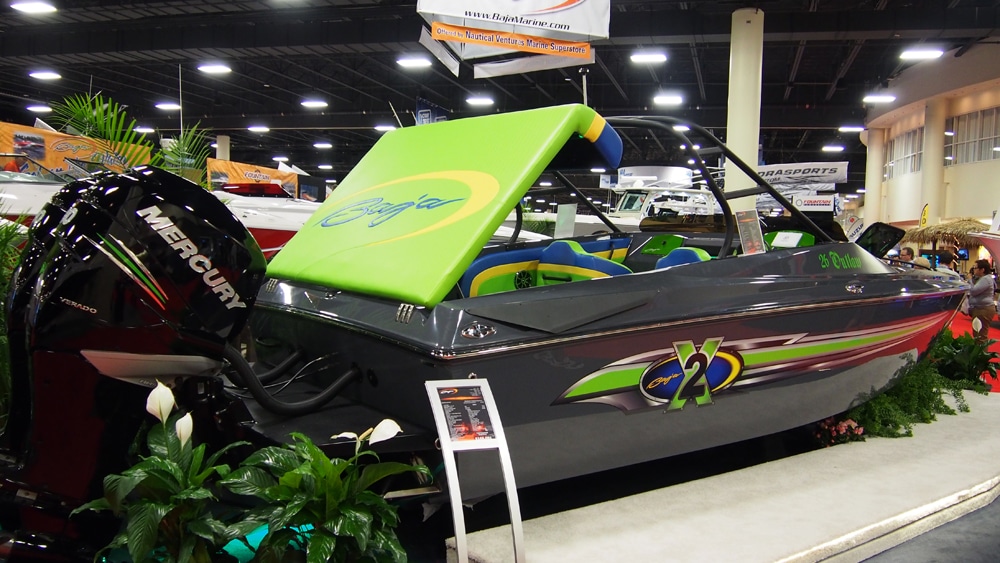In this detailed image of an indoor boat show, a sleek, medium-sized speedboat takes center stage within a large, well-lit hall featuring high industrial ceilings. The boat exhibits a striking combination of colors: a dark gray hull, a large green pinstripe running horizontally along its side, and an interior with vibrant blue, lime green, and yellow seating. The design also includes an 'X' with the number two on the side. The boat is powered by two large black Mercury engines at the back, each adorned with the brand’s name in vertical silver lettering and accented with green and silver pinstripes.

Surrounding the boat are lush green plants and white flowers arranged in potted displays, enhancing the aesthetic contrast. In front of the boat, a silver sign with details about the speedboat can be seen, but the text is not legible. The broader scene reveals other boats in the background, including a larger red and white vessel across from the featured speedboat. Orange and sports-related signage can be observed on the walls in the background, adding to the lively atmosphere of the showroom. The right side of the image reveals a windowed area providing a glimpse of the expansive boat show beyond.